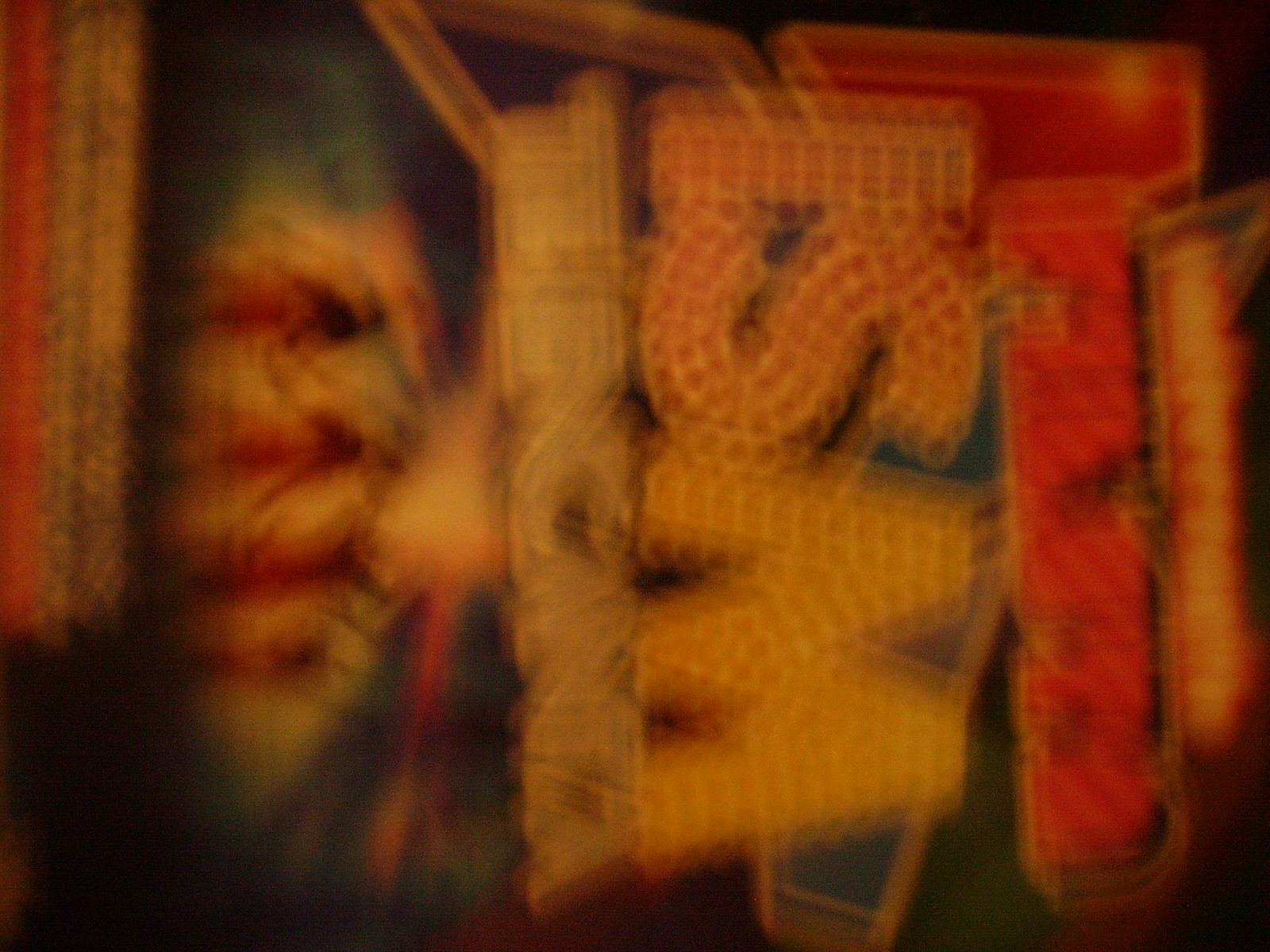The photograph shows an out-of-focus, blurry image of a brightly lit sign at night. The sign is rotated 90 degrees to the right, making the letters appear at an angle. Despite the blur, the sign's bold letters and vibrant lights are visible. The illuminated text features a mix of red, yellow, and green lights, creating an eye-catching display. The top text, though difficult to make out due to the blurriness, appears to be composed of yellow and red letters. The most prominent part of the sign displays the capital letters "ISM" in a striking manner. Below these letters is another word in blue text, followed by an indistinct image, adding to the sign's allure but making it challenging to determine its exact content.